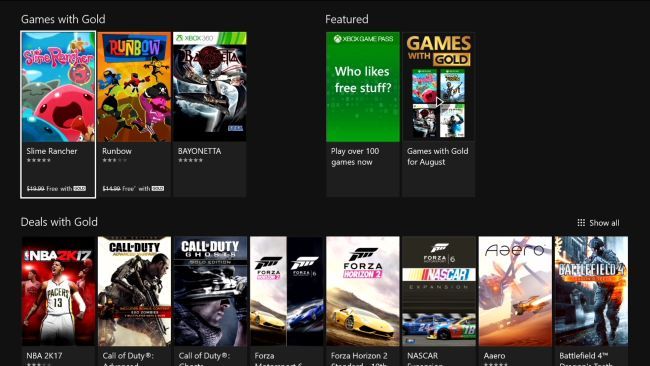The image depicts a black-screen interface showcasing a series of video games available for play. In the upper left-hand corner, the title "Games with Gold" is prominently displayed. Below this title, there are various cartoonish blob-like characters with exaggerated mouths, adding a playful element to the screen. Among the listed games, "Slime Rancher" stands out with a highlighted rectangular border, indicating its selection. Other games listed include "Runbow" and "Bayonetta." 

On the right side of the screen, there's a section titled "Featured" accompanied by a green "X" symbol, likely representing Xbox, and a tagline that reads "Who Likes Free Stuff?" Further to the right, additional "Games with Gold" are showcased.

Underneath the "Deals with Gold" section, the image displays a variety of popular titles, such as "NBA 17," "Call of Duty," "Forza," "NASCAR," "Aero," and "Battlefield." These games are available for play either online or on a computer, providing a diverse array of gaming options for users.